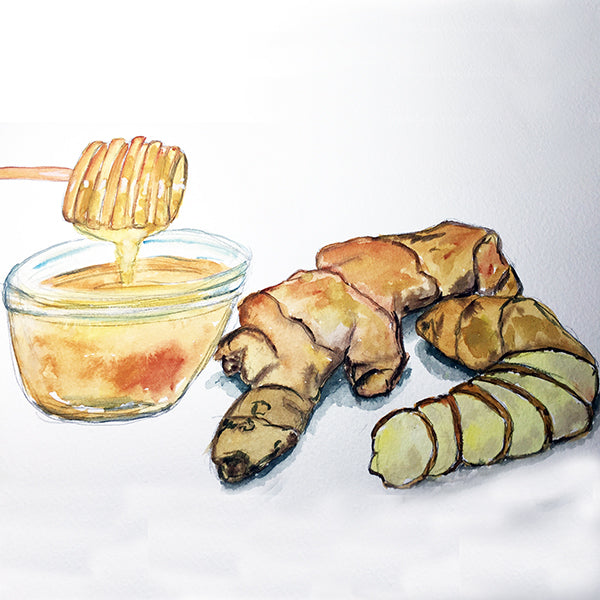The image is a square, possibly a painted piece with a predominantly blue background that transitions into white towards the bottom right and left edges. In the center left, there is a clear glass bowl filled with a yellowish liquid, likely honey, given that a honey dipper is positioned above it, dripping honey back into the bowl. The honey dipper, with its distinctive concentric grooves, has a slender handle and is partially out of frame on the left. To the right of the bowl, there are two brown objects. The first object, resembling a poorly illustrated piece of bread, is sectional with darker spots and lining, while the second object below it has a semi-circular shape, reminiscent of a crescent roll, featuring a segmented brown top and lighter sections on its curved side. The overall background integrates lighter shades, with areas of white, light gray, and hints of purplish hues, providing a neutral backdrop to the scene.